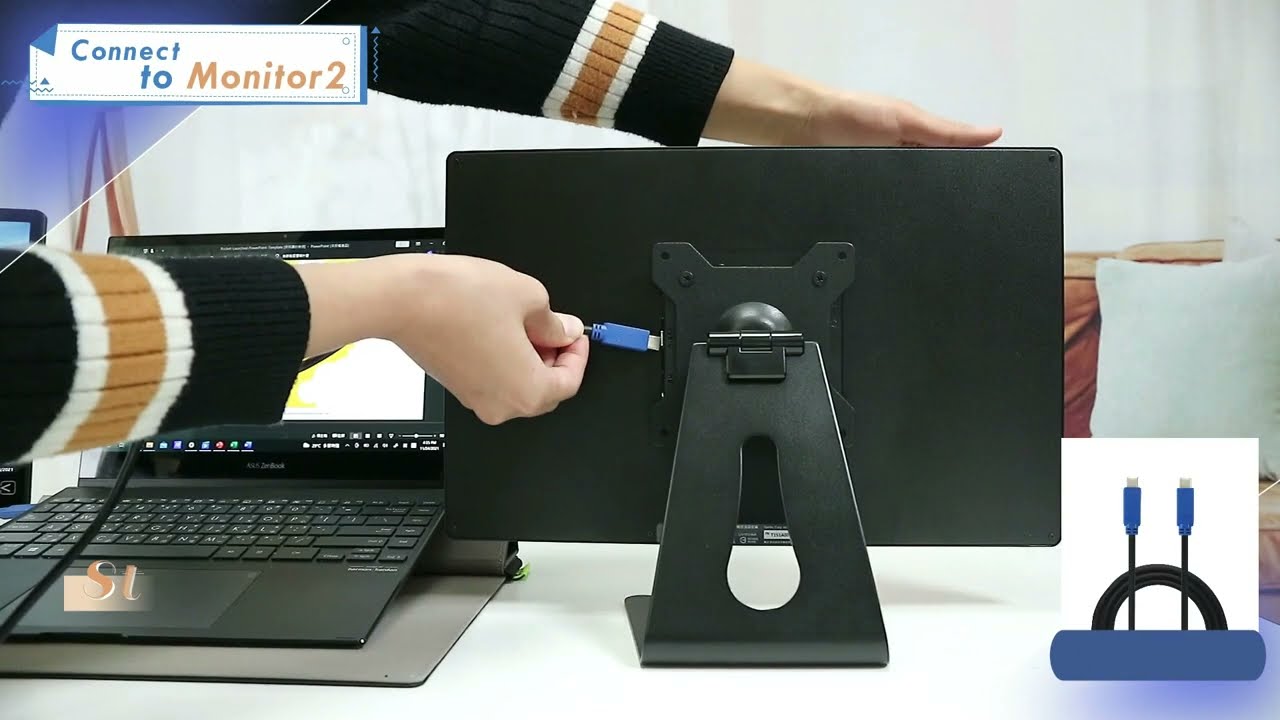The image features a detailed step-by-step demonstration of connecting a laptop to an external monitor. The main scene shows a person wearing a black sweater with white and brown bands around the wrist, plugging in a black cable with a blue end into the back of a monitor, which is facing away from the viewer. The black laptop, positioned on the left side of a white desk, is also connected to the cable. The laptop screen, partially obscured by the person's arm, displays the text "Connect to Monitor 2" on the top left corner. In the bottom right corner of the image, there's a small white box showcasing a product shot of the cable, suggesting it might be a micro USB, USB-C, or a similar type. The background includes a couch and a pillow, indicating a casual, possibly home setting, adding to the impression that this could be part of an educational tutorial or a product demonstration session.